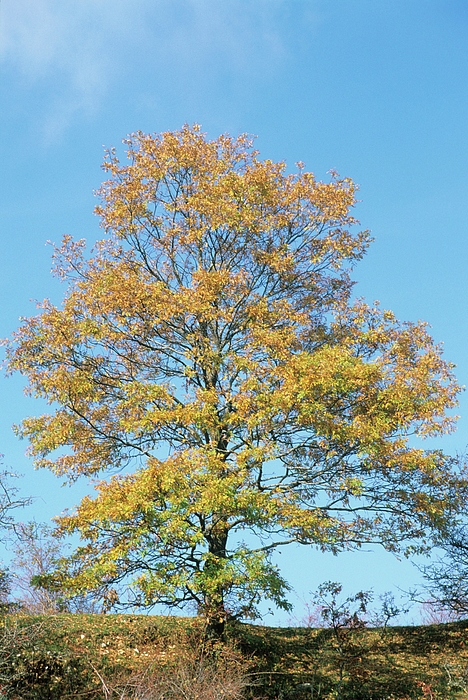This outdoor photograph captures a single tree set against a bright, cloudless blue sky, with sparse clouds only visible in the upper left corner. The tree, adorned with yellow leaves indicating the fall season, has its sparse foliage mostly concentrated at the branch edges. The mostly dry ground beneath is dotted with dry weeds, sticks, and leaves, and features very little grass. In the bottom right corner, you can faintly make out the outlines of another bare tree or bush. Shadows are cast on the ground in front of the tree. The camera appears to be positioned approximately 10 meters away, framing the image vertically ('hot dog way') to capture the entirety of this solitary tree in the dry landscape.